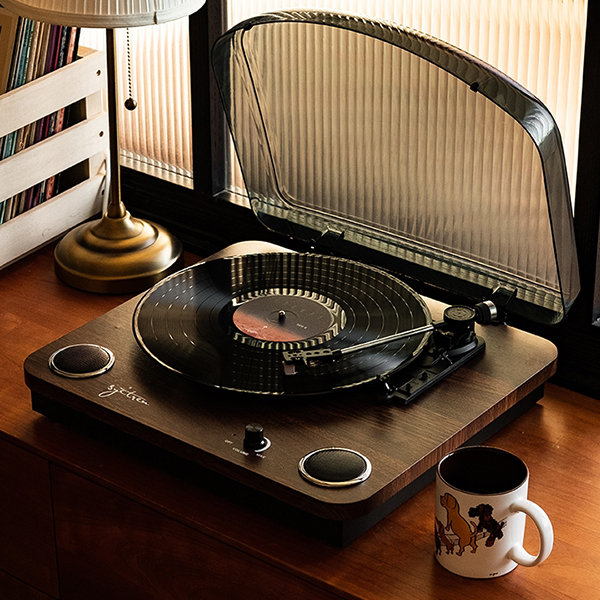This photograph features a vintage-style record player with a deep brown, wood-grained base and a clear, translucent cover that flips up. The cover appears to have a bronze tint. The record player, currently in operation, holds a black vinyl record with a black and red center. The metal needle arm, equipped with a black tip and base, is set on the record. Two circular speakers and a black volume knob are visible on the front of the wooden base. Positioned on a wooden desk or perhaps a cabinet, the setup is flanked by a lamp with a brass base and a white lampshade on the left and a white coffee mug with images of three dogs—one black, one tan, and one brown—on the right. To the left of the lamp, a wooden crate filled with music albums sits nearby. The background reveals beige window blinds against a darker window frame with black panes.